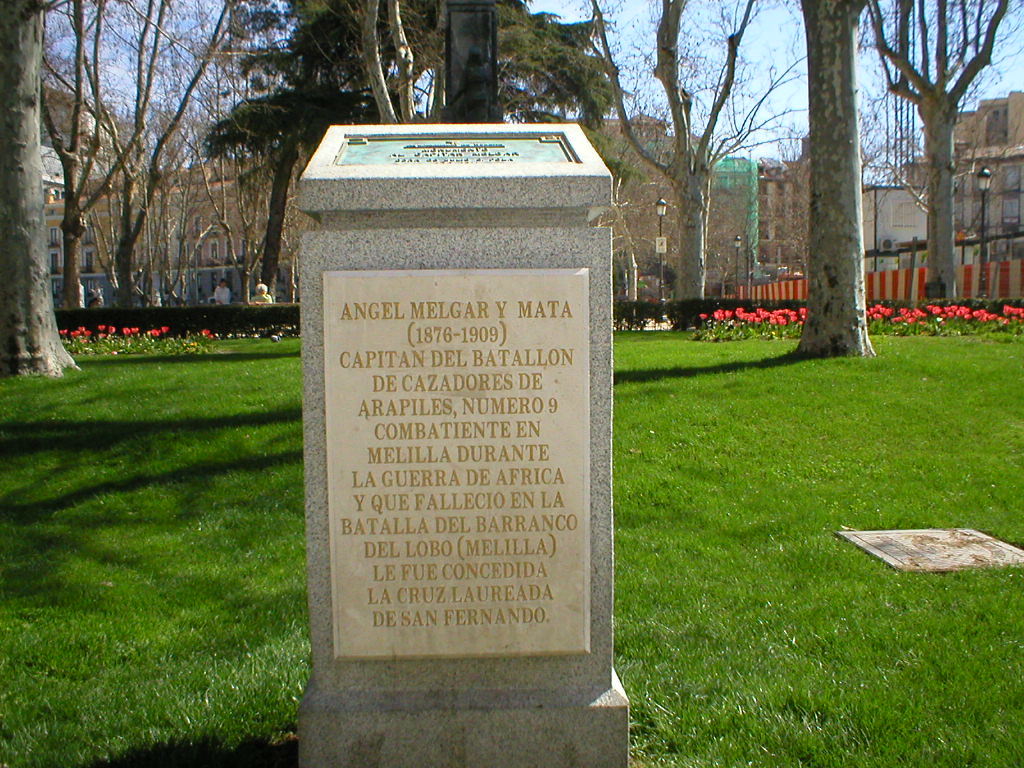This image captures a serene and meticulously maintained cemetery with a large, prominent gray headstone at the center. The headstone, which features a white faceplate with gold inscriptions, commemorates Angel Melgar Guaymata, who lived from 1876 to 1909 and was a captain of the Battalion of Cazadores de Arapilis, Number 9. He fought in Melilla during the War of Africa and fell in the Battle of Barranco del Lobo, earning the Arid Cross of San Fernando.

The headstone stands amidst a lush, expansive field of well-manicured, vibrant green grass that stretches from the middle to the bottom of the image. In the far background, flower beds with red and pink flowers add pops of color, flanking either side of the scene. Numerous tree stumps and bare tree trunks populate the middle background, with one tree displaying some green foliage.

Beyond the trees, parts of several buildings, possibly apartments, are visible, including a brown brick structure partially obscured in the distance. Additionally, a worn, gray and brown flat stone lies in the grass to the right of the main headstone, reinforcing the cemetery setting of this peaceful landscape.